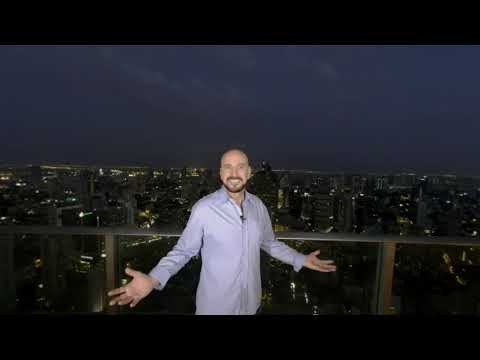In this nighttime photograph, a bald or shaved-headed Caucasian man with a brown mustache, brown beard, and goatee stands smiling broadly on a high balcony overlooking a sprawling cityscape. He is dressed in a long-sleeve, blue button-up shirt, and his outstretched arms and upturned palms suggest a joyful, "here I am" gesture. The glass-paneled railing behind him reaches the middle of his back, emphasizing the height of the platform. The darkening sky, a deep midnight blue, forms the backdrop, dotted with city lights just beginning to illuminate the numerous buildings and structures below. His jubilant expression and open stance capture a moment of pure enjoyment against the beautiful urban panorama.